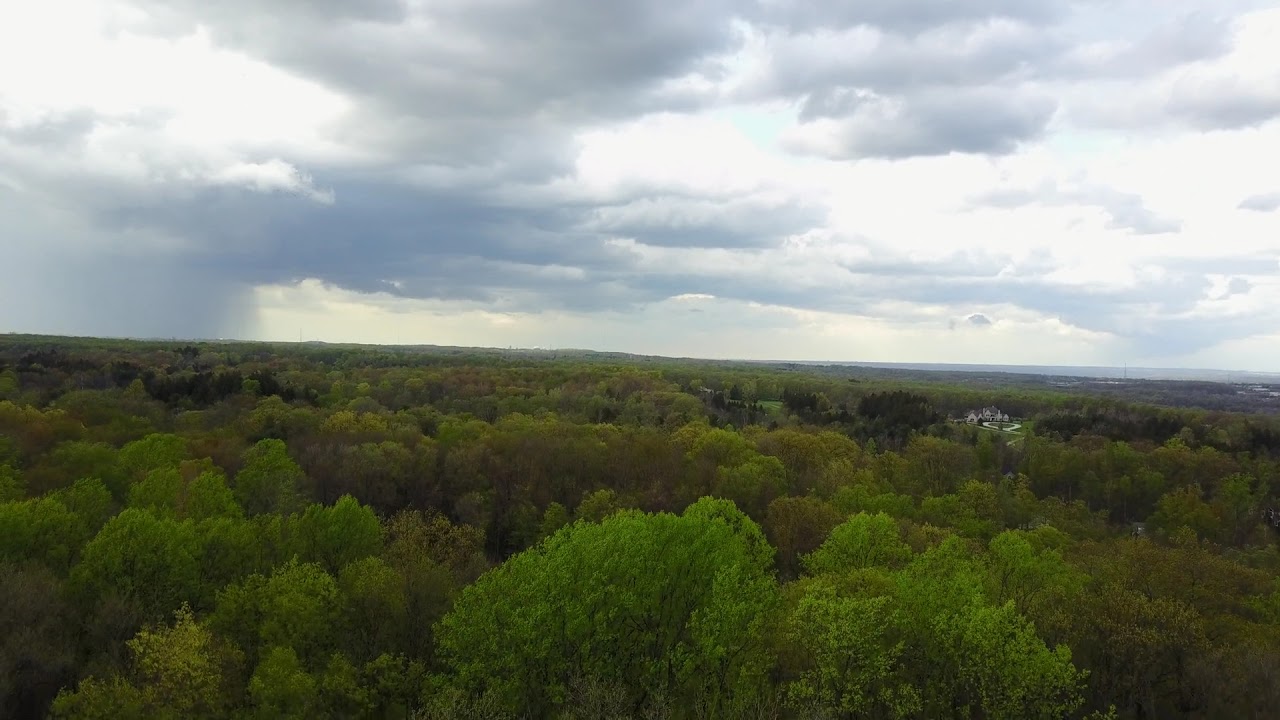This detailed aerial, landscape-orientation color photograph captures an extensive forest, sprawling with bright green trees transitioning to deeper greens and browns. The densely wooded area extends to a flat horizon, under a heavily overcast sky with dark storm clouds hanging ominously, although some sunlight struggles to pierce through. Nestled in the middle-right of the image, partially concealed by treetops, is a large, gray estate with a dark roof and multiple connected wings, accessible via a white path. On the left side of the image, a rainstorm is visible under the gray clouds. The scene, likely early spring given the mix of vibrant greens and sparse, brownish trees, is captured from a high vantage point, probably by a drone, providing a comprehensive view of the forest and the distant beginnings of a town.